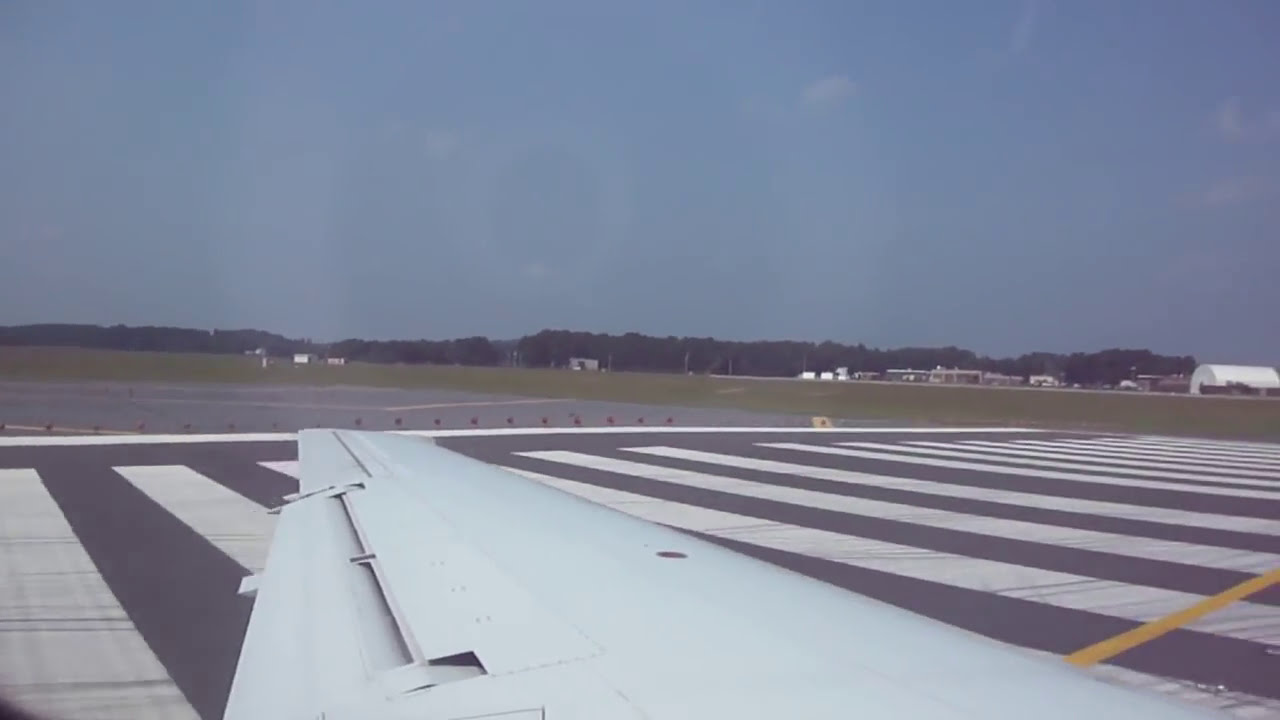The photo captures a detailed view from inside an airplane, looking over its large, white wing extending toward the distance. The foreground shows the wing prominently, while the person taking the picture is positioned next to the window. The image includes a clear, blue daytime sky with a slight haze and a few scattered clouds. In the distance, a runway is visible, adorned with several large, white rectangular stripes and a distinct narrow yellow line running perpendicular to them. Further along the runway, a prominent horizontal white stripe marks the area beyond which a series of unlit beacons or signal lights are situated. To the right, distant airport structures are noticeable, including a white airplane hangar and a smaller concrete building. The scene is complemented by surrounding grassy fields and a line of trees encircling the airport, with several trucks or planes faintly visible on the faraway tarmac. The upper portion of the photo showcases a dark blue sky, potentially with camera-related spots that somewhat resemble clouds.